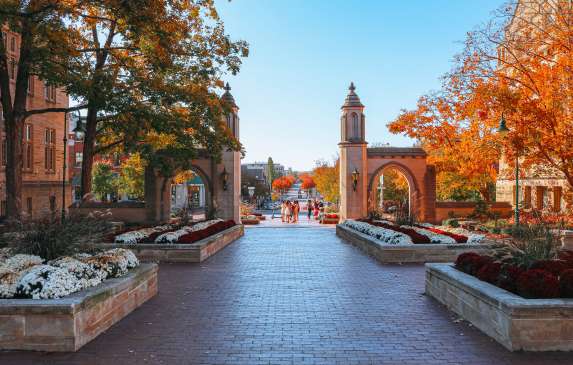The photo captures a serene courtyard, likely at a European university or church, characterized by its elegant and open architecture. Two brick arches form a grand entranceway, flanked by walkway towers with lamps. The pathway and nearby structures are constructed from reddish-brown brick, exuding an old-world charm. The courtyard itself is meticulously maintained, adorned with rows of white and red flowers. Vibrantly colored autumn trees, with golden and orange leaves, frame the scene on both sides. A big orange tree stands out to the right, while a yellowish-green one graces the left. The sky is a clear, beautiful blue, enhancing the tranquil atmosphere. In the distance, people can be seen strolling along the paved walkways, which further accentuate the peaceful and inviting ambiance of the area. The overall setting, with its lush flower beds, historical architecture, and serene environment, creates a picturesque and idyllic backdrop, perfect for a leisurely walk or quiet reflection.